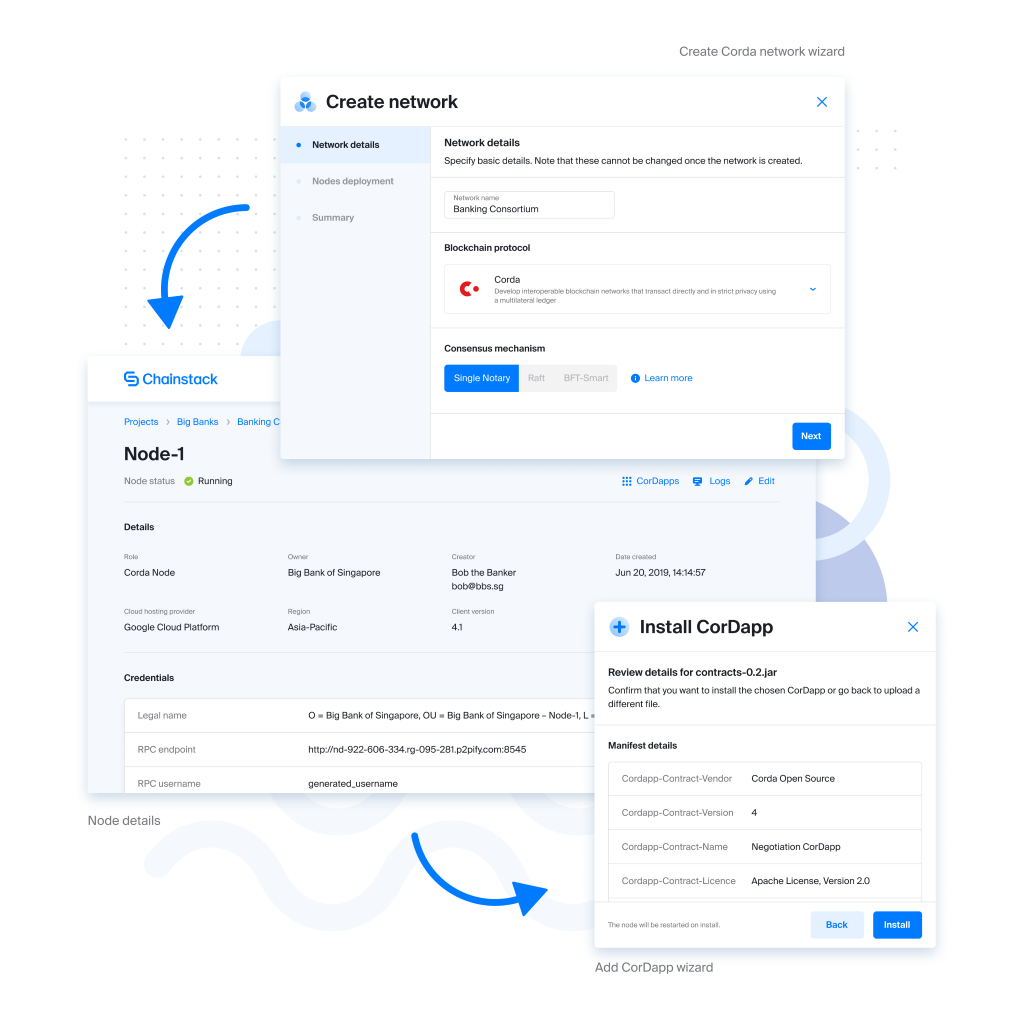**Caption:**

The image depicts a step-by-step diagram for setting up a blockchain network using Corda. 

- At the top, there is a label that reads "Create Network," setting the stage for the diagram.
- Below this title, three illustrated squares represent different functionalities, connected by a blue arrow that curves to the right and then downwards, guiding the flow of information.
- The first square, labeled "Network Details," is an introduction to the network setup.
- The second square, titled "Banking Consortium," indicates the involvement of multiple banking institutions.
- The third square, "Blockchain Protocol," specifies the usage of a blockchain system.
  
  Below these squares:

- There is a rectangle that points to the left, indicating a procedural step or additional information context.
  
Further down, there is another square labeled "Corda," followed by the subtitle "Consensus Mechanism." This section elaborates on three selectable mechanisms:
- "Single Notary," highlighted by a blue line, indicating it's the currently selected option.
- "RAH" (presumably another consensus option).
- "BFT Smart" (Byzantine Fault Tolerance).

Next, a separate section labeled "Chainstack" (presumably a service or tool related to the setup) is identified below the consensus mechanism options.

Lastly, the diagram concludes with a square labeled "Install Corda," indicating the final step for the network setup.

This detailed diagram visually guides one through the process of creating and configuring a network using the Corda blockchain platform, highlighting essential steps and choices within the setup workflow.